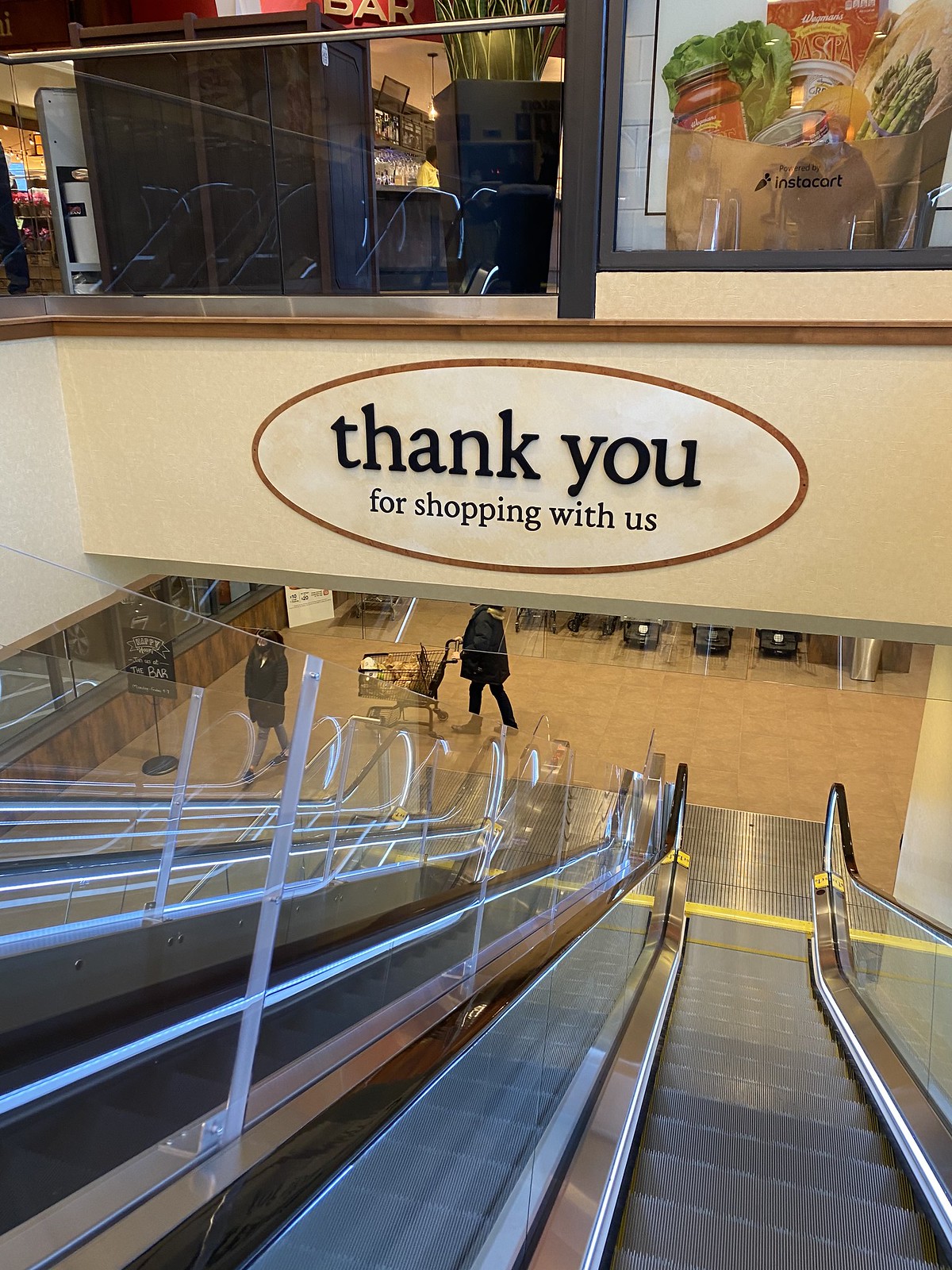A point-of-view photograph captures the scene from someone descending a silver and black escalator, likely located in a shopping mall. Prominently displayed above the escalator is an oval sign featuring large, dark black letters spelling out "Thank You." Beneath this, in smaller black letters, the sign continues with "for shopping with us." At the base of the escalator, just slightly to the left, a person is visible pushing a shopping cart, while another individual walks ahead of the cart. Above the "Thank You" sign, additional signage is observed, including an image of a grocery bag filled with various items such as lettuce, asparagus, and a jarred food item. To the left of this grocery-themed sign, there appears to be other display materials, though they are indistinct. The overall perspective of the image is from the viewpoint of someone looking downwards while riding the escalator.